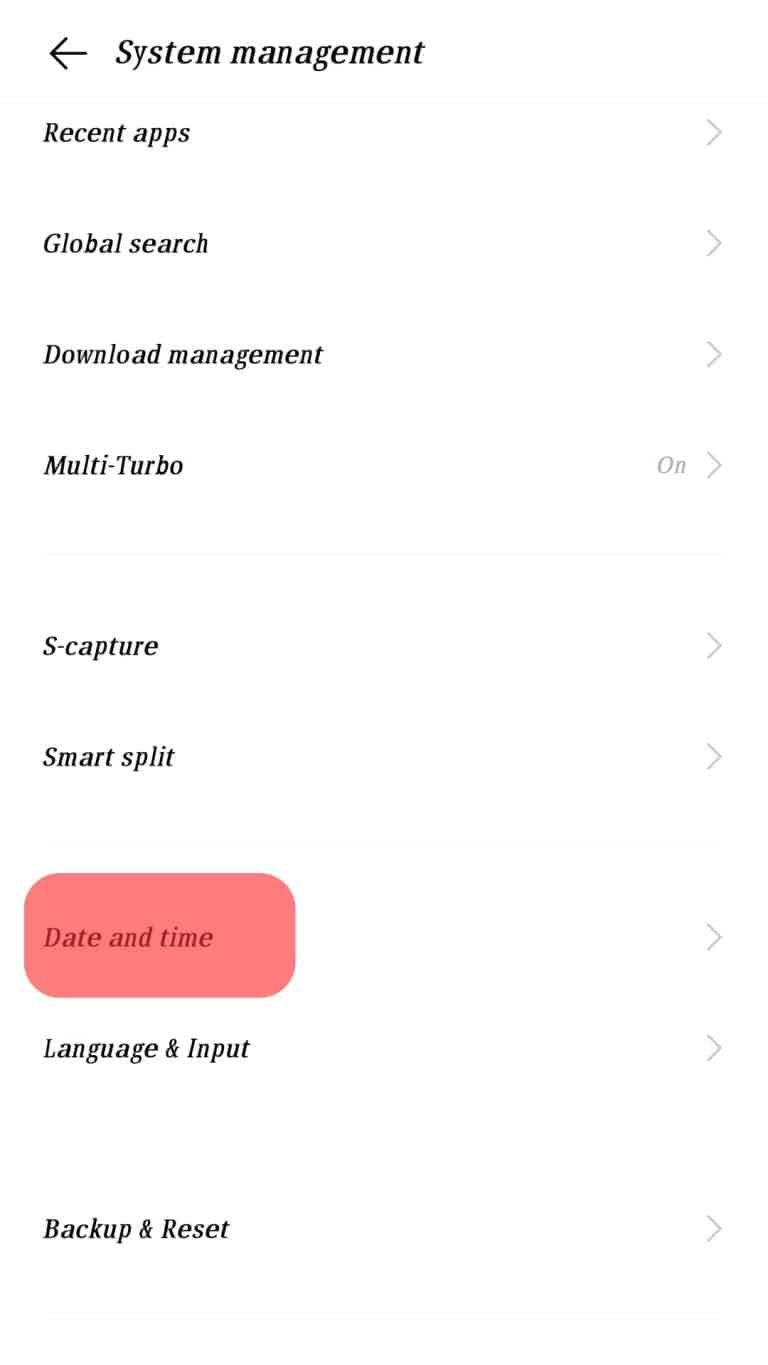Screenshot of a system management interface with various settings options listed. At the top, there is a black arrow pointing to the left next to the text "System Management." Below this title, a series of options are displayed, each with a right-pointing arrow indicating further details or actions. The options listed are: "Recent Apps," "Global Search," "Download Management," "Multi Turbo On," "S Capture," "Smart Split," "Date and Time," "Language and Input," and "Backup and Reset." Notably, the "Date and Time" section is highlighted with a pink rectangle featuring rounded edges. The layout is predominantly text-based with no photographic or graphic elements. The image is significantly taller than it is wide, providing a vertical list of settings options. The screenshot is devoid of any people, animals, plants, buildings, or vehicles.